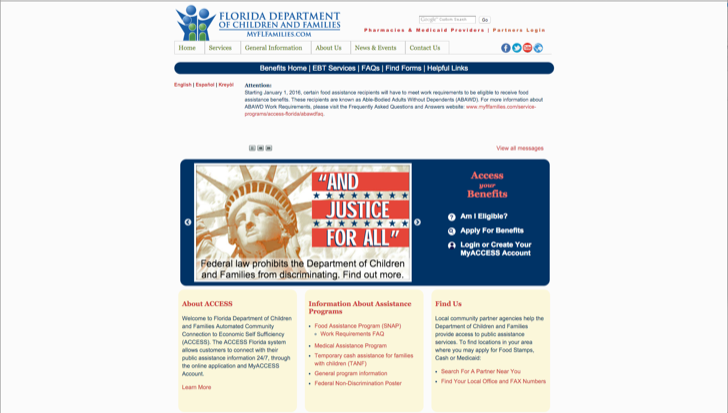The image displays a webpage with an off-white background and centered content. At the top, in blue text, it reads "Florida Department of Children and Families." Below that, a URL is partially visible, possibly "myflfamilies.com." Further down, it mentions "Pharmacies and Medicaid Providers/Partners League," although part of the text is unclear. 

The webpage features several tabs with white backgrounds and little squares. In green, it lists various sections: "Home," "Services," "General Information," "About Us," "News and Events," and "Contact Us." Social media icons for Facebook, Twitter, YouTube, and an unidentifiable blue symbol are also present.

A blue oval contains white text that includes "Benefits Home," "EBT Services," "FAQs," "Forms," and "Helpful Links." Underneath, in red text, it says "English," "Español," and an unreadable third language.

A red alert message reads: "Attention: Starting January 1st, 2016, certain food assistance recipients will have to..." with the rest of the text blurred and illegible. Below this, another red message states "Access Your Benefits," followed by options to "Am I eligible to apply for benefits?" "Log in or create your My Access account." Additionally, there are links for "About Access," "Information about assistance programs," and "Find Us."